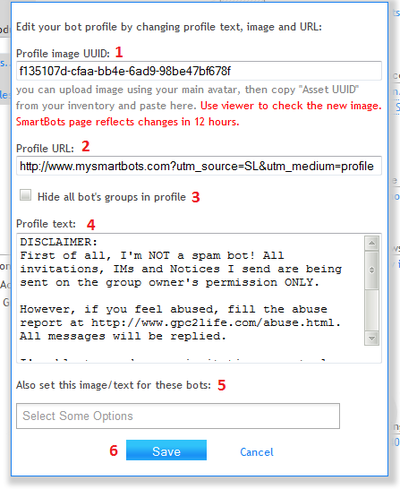This detailed caption describes a pop-up window related to bot profile editing in what appears to be a technical context, possibly involving coding or software development.

---

The pop-up window for editing a bot profile is prominently displayed, offering several options for customization. The first line instructs users to "Edit your bot profile by changing profile text, image, and URL." Directly below, the instruction "Edit profile image UUID" is highlighted with a red number 1. 

A search bar underneath contains a serial number, and an informative note states that users can upload images via their main avatar and then copy the asset UUID. Another highlighted reminder in red advises users to "use viewer to check the new image. Smart bots page reflects changes in 12 hours."

Following these instructions is a designated profile URL field with a red number 2 beside it, accompanied by an address bar. Additionally, there's an option to hide all bot groups in the profile, marked with a red number 3.

Situated at the bottom of the window is a profile text box, indicated by a red number 4. Adjacent to this is a scrollable white box containing a disclaimer: 

"First of all, I'm not a spam bot. All invitations I am to notices I send are being sent on the group owner's permission only. However, if you feel abused, fill the abuse report at www.gpc2life.com/abuse.html. All messages will be replied to."

The final line in the window includes the instruction "set this image/text for these bots," tagged with a red number 5. Below this line is a search bar, and to the right, a blue save button marked with a red number 6, accompanied by a cancel link.

---